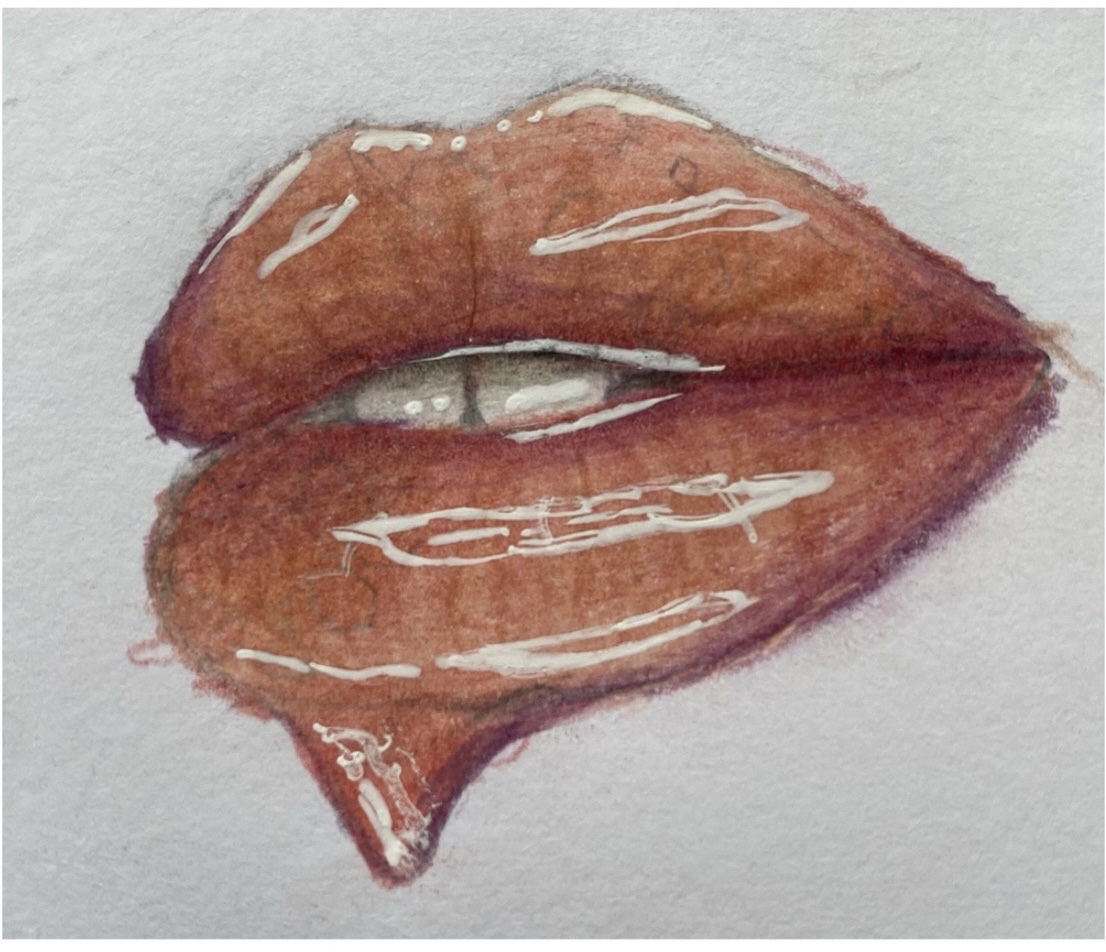This color image depicts an art piece of a sketched and painted pair of glossy, plump lips in a light reddish-pinkish coral hue, set against a completely white background. The lips are slightly parted, revealing the top two front teeth. The artwork seems to have been initially drawn with pencil and then richly colored, possibly with colored pencils or paint, giving the lips a highly reflective, almost varnished appearance. There are strategic white highlights on and around the lips, enhancing the glossy effect, while some darker purplish-red outlines and charcoal pencil marks are visible, suggesting an unfinished look. Additionally, there appears to be a drop of red, resembling blood, dripping from one corner of the mouth, adding an intriguing and dramatic element to the piece.